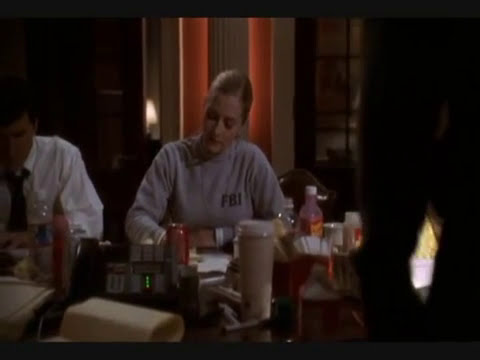The image appears to be a still from a movie, featuring a scene inside a room. Central to the image is a blonde-haired woman dressed in a gray full-sleeve t-shirt with "FBI" written on it. She is seated at a large table cluttered with various items including bottles, papers, and what seems like a Pepto-Bismol bottle, indicating a work environment, possibly a conference table. The woman is looking down, apparently writing or taking notes on the papers in front of her. To her left, partially cut off by the frame, is a man wearing a white shirt with a loosened black tie, also looking downwards. The background features two red pillars, adding to the ambiance of the room. The right side of the image fades to black, with the lower right-hand corner displaying what seems to be a torch. Overall, the scene suggests a serious, work-focused atmosphere.